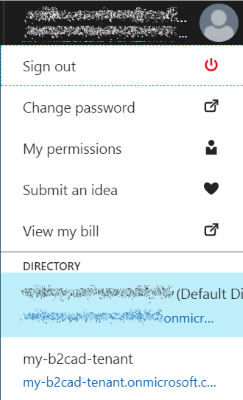The image is a screenshot of a phone application with a black header at the top. This header has most of its contents obscured by irregular shapes resembling snowflakes or salt, creating an abstract blockage. To the right within this header is a generic profile icon depicting the outline of a person.

Below the header, there is a "Sign Out" option in white text, underlined by a dotted blue line, accompanied by a red power button icon with a circle around a dash positioned at the top center. Directly below this line, there are several options listed:
- "Change Password"
- "My Permissions"
- "Submit an ID of You"
- "My Bill"

Following these options is a series of icons: what appears to be a "Pop-Out" option, a "Torso" icon (perhaps representing user profile settings), a "Heart" icon (potentially for favorites or likes), and another "Pop-Out" option.

Next, a solid line separates the previous section from the subsequent "Directory" label, below which is a blue field with more contents scribbled out similarly as before. The first obscured line includes a partially visible bracket that reads "default DI..." and is cut off. The second line shows a partial text, "onmicr...", on the right side of another scribbled area.

Continuing down, in a white field, the text "my-b2cad-tenant" appears, followed by its smaller, blue-text counterpart "my-b2cad-tenant.ommicrosoft.c...". A solid black line, only one pixel in width, runs vertically along the left side of the screenshot. The entire layout presents a somewhat cluttered and obscured interface with various sections and labels partly hidden.